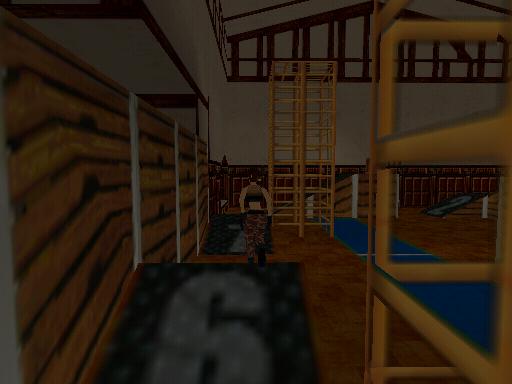This screenshot, taken from a low-quality, dark video game with 64-bit graphics, depicts the interior of a building. To the left, there is a wooden wall, while a white wall with two ladders leading up to windows is positioned centrally. In the middle of the scene, a small soldier-like character is walking. Dominating the forefront is a black box marked with the number 6 in gray. To the left, yellow bunk beds are visible, and a large box with the number 2 is situated on the right. The floor features a wood grain texture, contributing to the overall setting's rustic appearance.